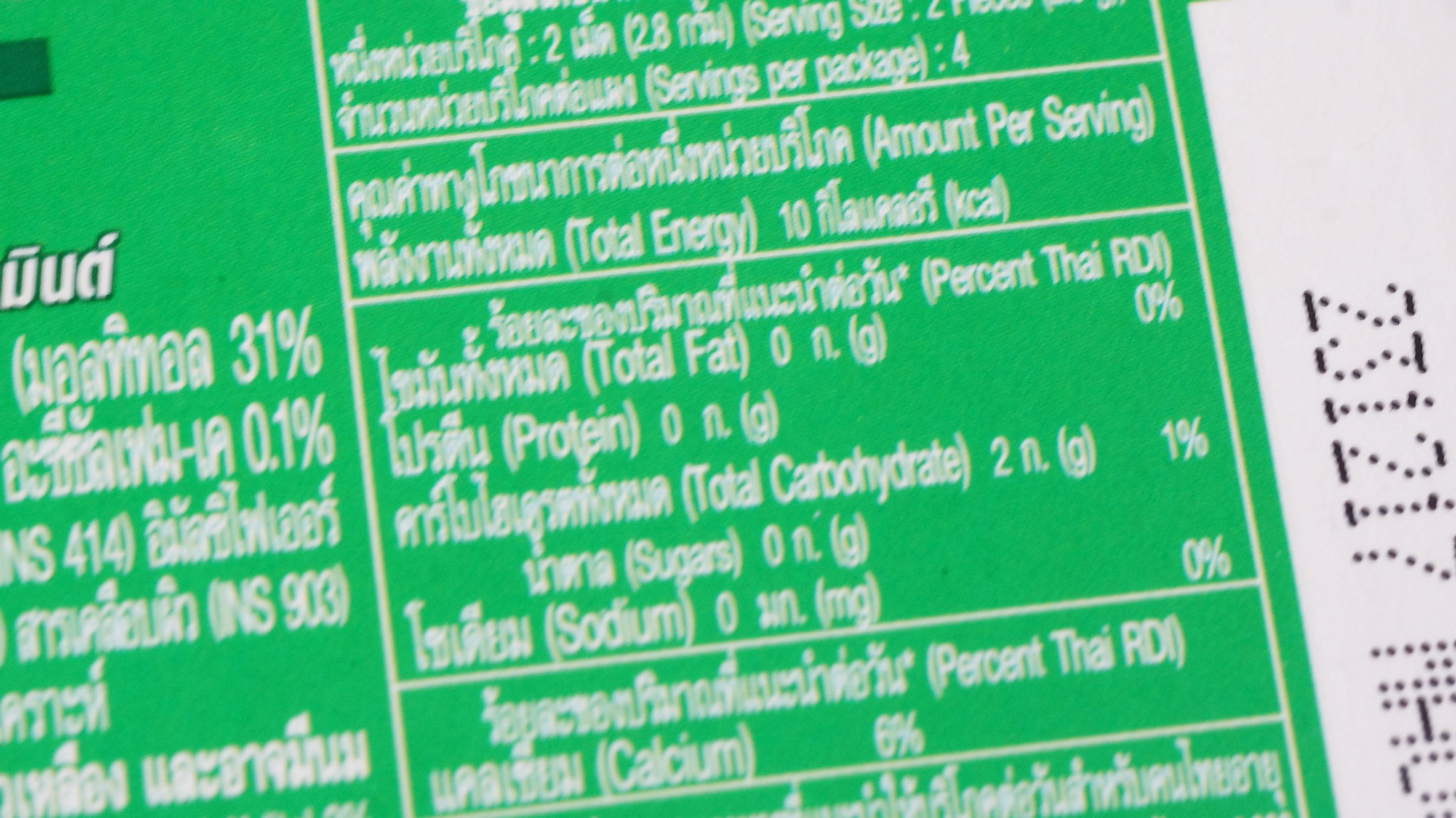The image shows a close-up of a nutritional label on the back of a kelly green package. The label features white font divided into sections by white lines and includes both a foreign language—likely Thai—and English translations in parentheses. It lists the nutritional information per serving, with the package containing 4 servings. The details include total energy (10 units), protein (0%), total fat (0%), carbohydrates (1%), sodium (0%), and calcium (6%). On the right edge, there are numbers and letters printed in a dot matrix style: "231217 MHO," which could be a product ID or expiration date, tilted slightly to the left.